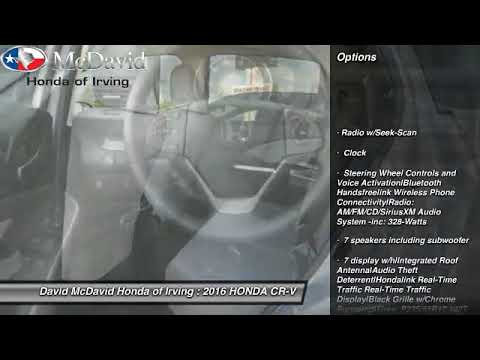The image is a detailed advertisement for a 2016 Honda CR-V from McDavid Honda of Irving. The background is a grayscale, semi-transparent overlay showing both the backseat and steering wheel of the vehicle, creating a transition effect. In the upper left corner, there's a Texas flag icon with the state of Texas superimposed on it, along with silver gradient text reading "McDavid" and black text below that stating "Honda of Irving". The bottom portion of the image reiterates the dealership's name and the vehicle model. On the right side, white text on a black transparent background lists various car options, including a radio with seek scan, clock, steering wheel controls with voice activation, Bluetooth hands-free link, wireless phone connectivity, and an advanced audio system with 325 watts, 7 speakers including a subwoofer, a 7-inch display, integrated roof antenna, and an audio theft deterrent feature. This text appears in bullet points but fades out towards the end, making the last few details somewhat difficult to read.